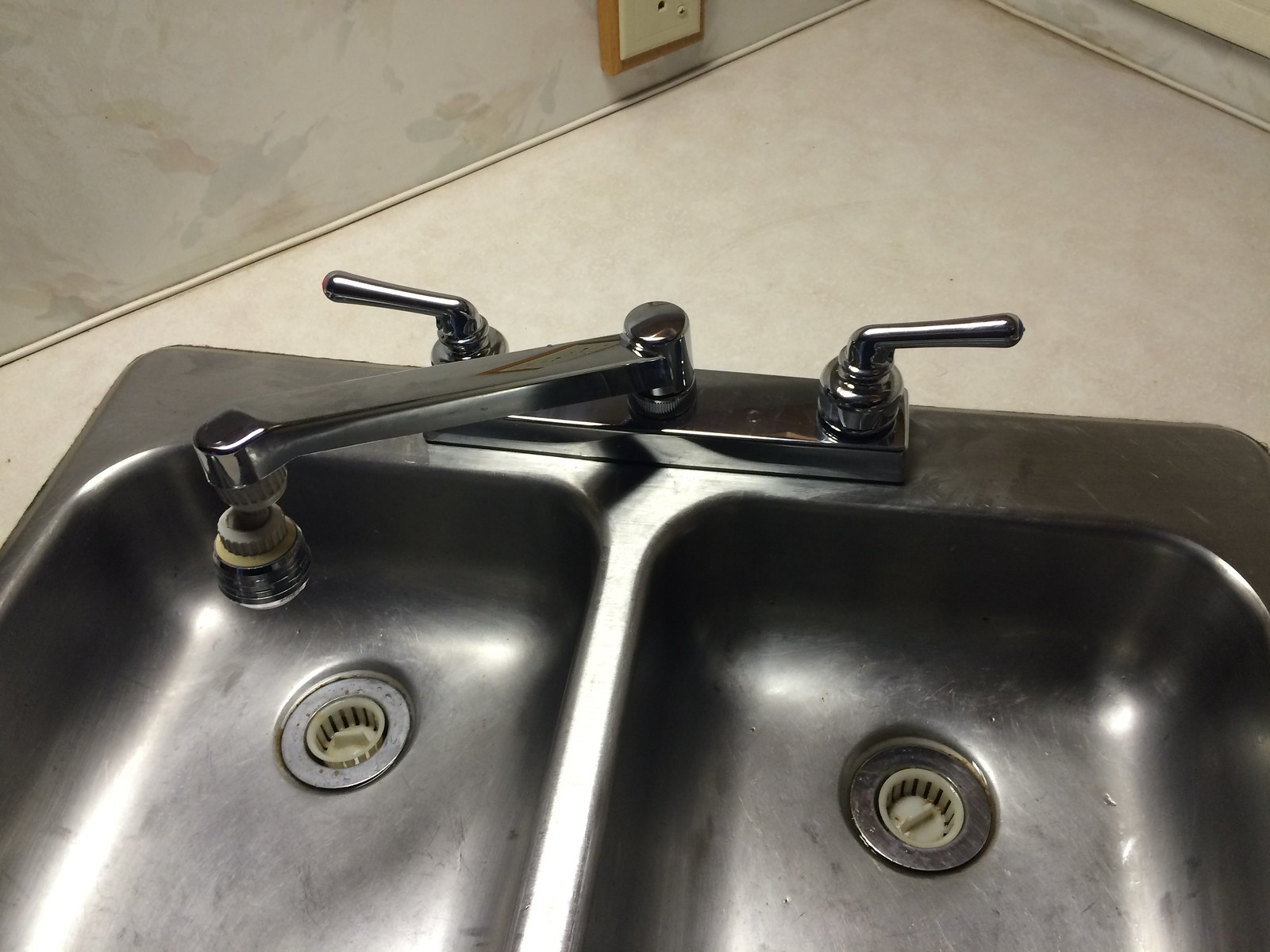This photograph features a double-sided stainless steel kitchen sink set into a whitish beige countertop in a corner. The wall in the background is also a whitish beige with streaks of pale gray and beige, and a portion of an outlet mounted on a wood block is partially visible. The sink, showing signs of wear and scratches, is equipped with two white plastic strainers in each drain to filter out food or other debris. Drops of liquid can be seen on the right side. The faucet, made of shiny chrome, arches over the left side of the sink and has two horizontal handles with rounded ends for controlling the water flow. The sturdy, metallic faucet can be moved from left to right, and the area near the sink includes a marbled counter surface adding to the kitchen's corner aesthetic.